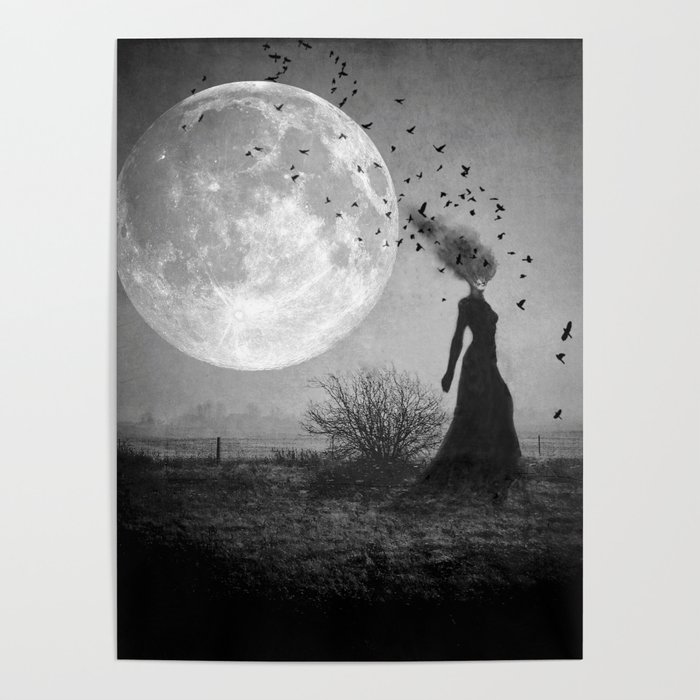This eerie black and white image captures a haunting outdoor scene under a large full moon that occupies the top quarter of the frame. The moon, detailed with craters, casts a ghostly glow over a desolate field. In the distance, the outline of a fence can be seen behind a leafless bush. Dominating the right side of the image is the silhouette of a tall woman in a long black gown with long sleeves or possibly black gloves. Her face is obscured and blends into a surreal gray plume, resembling either hair or smoke, that stretches towards the moon. A large flock of black birds or bats is seen flying around her and across the moon, enhancing the ominous atmosphere of the scene. The entire composition is steeped in dark, haunting shades, adding to its ethereal quality.